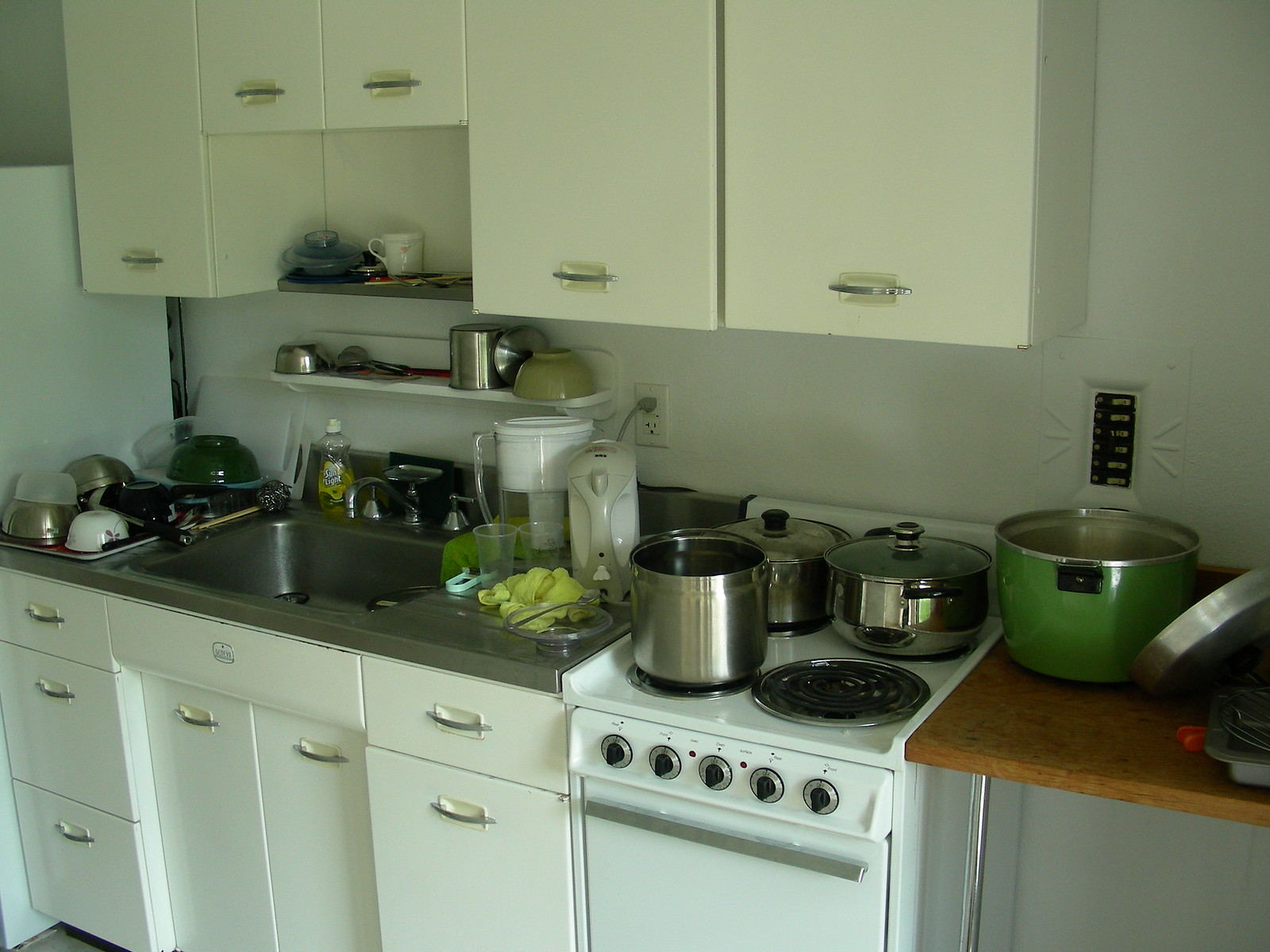In this image, a partial view of a kitchen is captured, focusing on the area around the sink and stove. The compact, white stove stands out as unusually small compared to typical household stoves, with three pots resting on its surface. To the left of the stove, the counter holds a few items, including a pitcher, a clear plastic cup, and a yellow rag. The sink is located further to the left, accompanied by a stack of dishes piled up on its side. Above the sink, two shelves are visible, holding a coffee mug and a silver object. Surrounding the scene, white cabinets offer a clean and cohesive look, while to the right of the stove, there is a green bowl adding a splash of color to the otherwise monochromatic setting.